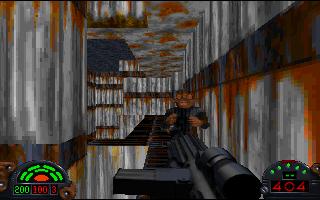In the video game screenshot, the bottom left corner prominently features an emblem showcasing "200" in green text, followed by "100" in red. Adjacent to it is a red "3" encased within a gray border, accompanied by green curved lines that encircle an orange oval shape. To the right of this emblem, an icon displaying "404" in red text is visible, topped by five green lights and set against a gray platform.

Dominating the lower portion of the screen, a black gun is positioned sideways, allowing a clear view of its magazine and scope. The character in the foreground is brown and distinctively marked by three brown eyes on its face. The overall scenery is predominantly light gray, smeared with numerous orange stains, contributing to a gritty atmosphere. The walkable platform at the bottom is black, contrasting with the setting. Additionally, a solitary black square can be seen on the ceiling, adding an element of symmetry to the environment.